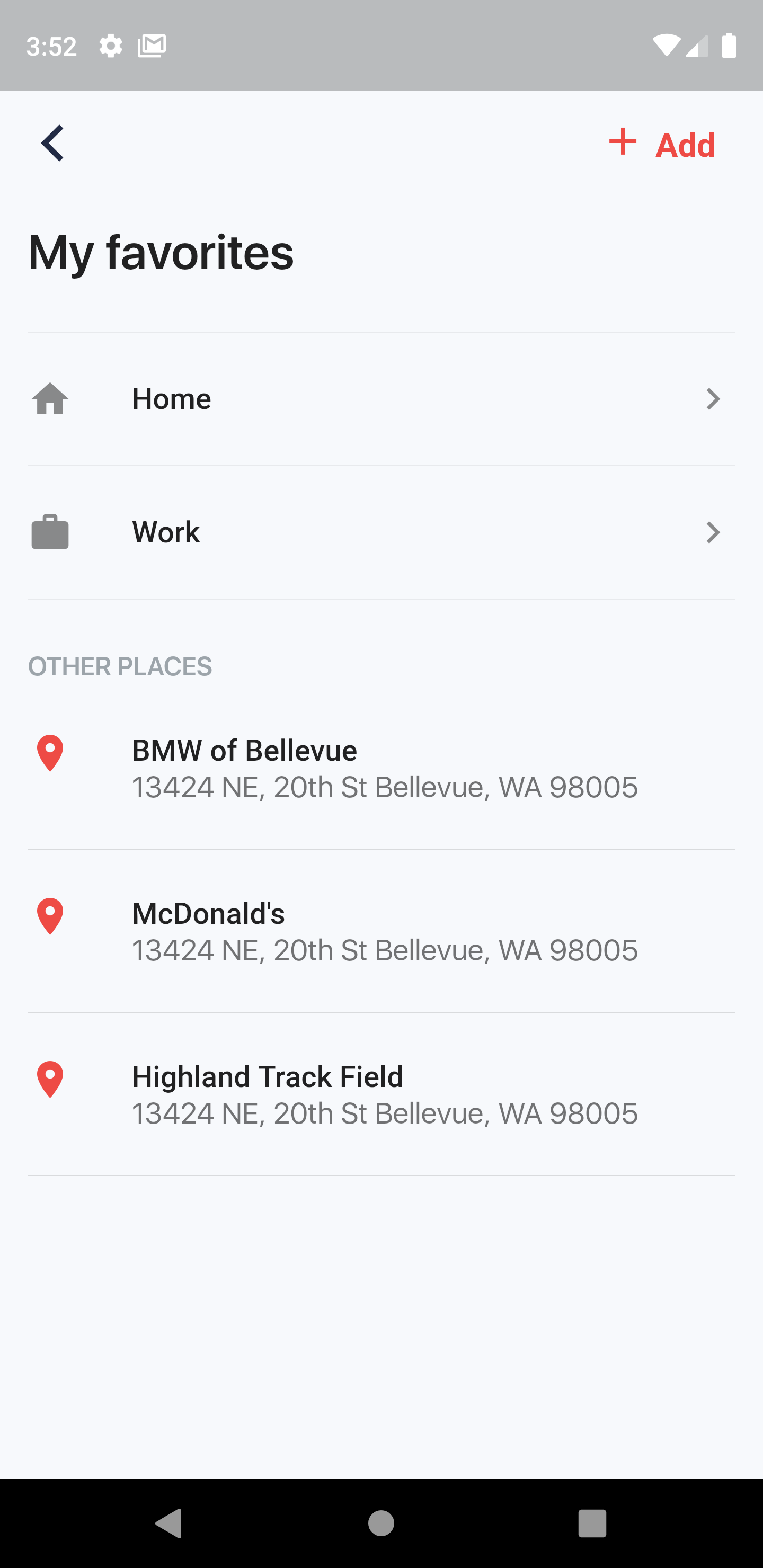This image is a detailed screenshot of a phone's "My Favorites" section, highlighting preferred places. The time shown is 3:52. The phone has a notification indicating pending messages, Wi-Fi is enabled, the signal strength is at half bars, and the battery appears almost full.

At the top, there's a navigation bar featuring a back button on the left, a red plus sign, and an "Add" button. The section title, "My Favorites," is prominently displayed in black text.

The list includes:
1. **Home** - with a context menu for further options.
2. **Work** - also with a similar context menu.

Additionally, there is a segment labeled "Other Places," showcasing three entries marked by upside-down rounded triangle place markers with white dots:
1. **BMW of Bellevue** - Located at 13424 Northeast 20th Street, Bellevue, Washington, 98005.
2. **McDonald's** - Also at 13424 Northeast 20th Street, Bellevue, Washington, 98005.
3. **Highland Track Field** - Situated at the same address: 13424 Northeast 20th Street, Bellevue, Washington, 98005.

The textual information is presented in black on a white background. At the bottom of the screen, there's a black navigation bar with icons for back, home, and menu.